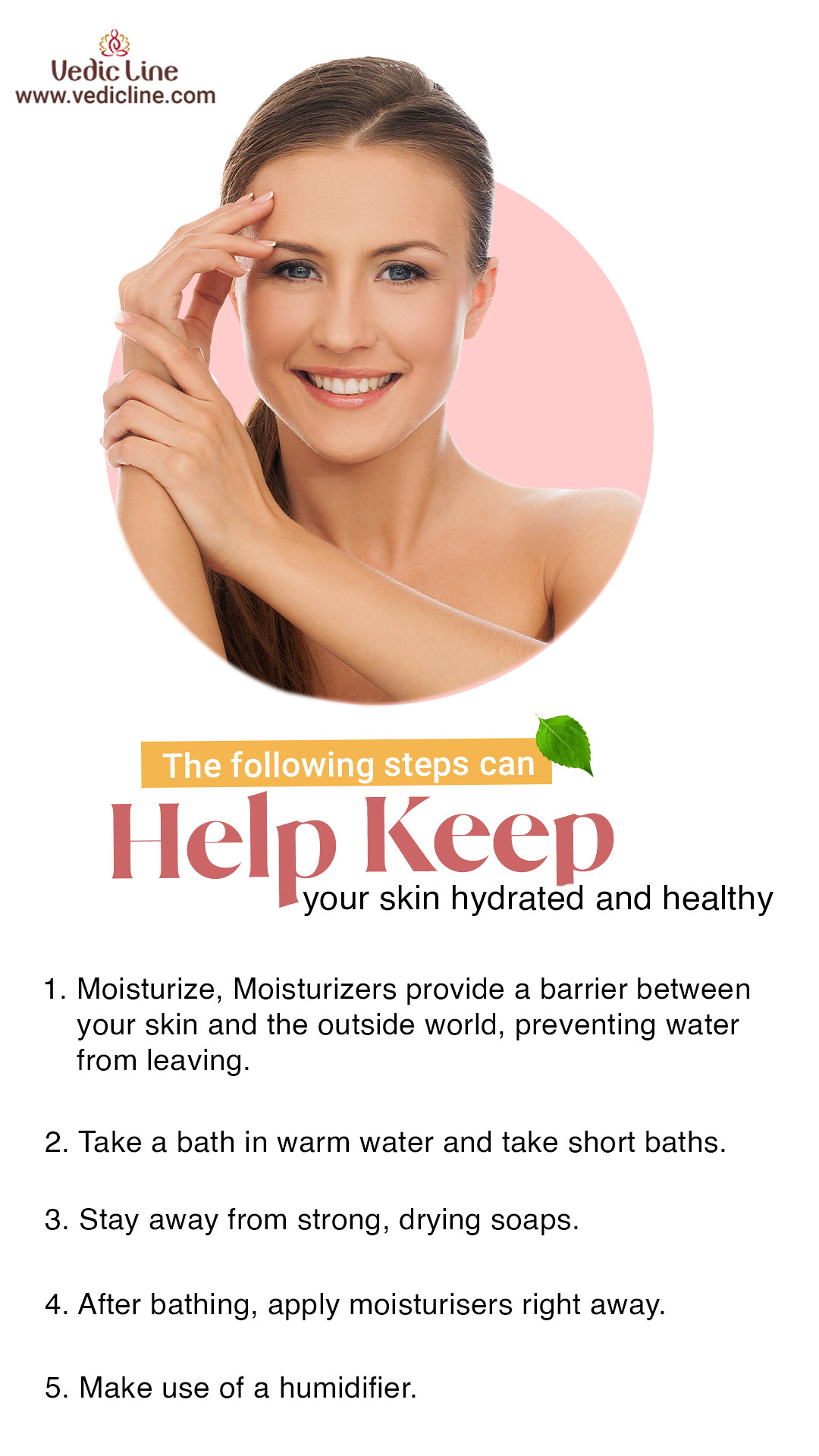The advertisement for Vedic Line (www.VedicLine.com) features a portrait of a smiling woman with brown hair cascading down to her chest. She is looking directly into the camera, displaying her upper set of teeth. Her pose includes her left hand gently touching her right wrist and her right hand resting on the side of her head. Positioned on a simple white background, the top left corner displays the Vedic Line logo. Below the portrait is a list titled "The following steps can help keep your skin hydrated and healthy," featuring these steps: 1. Moisturize. Moisturizer provides a barrier between your skin and the outside world, preventing water from escaping. 2. Take short baths in warm water. 3. Avoid strong drying soaps. 4. Apply moisturizer immediately after bathing. 5. Use a humidifier. There is a green leaf icon in the middle of the image, adding a touch of freshness to the overall aesthetic.